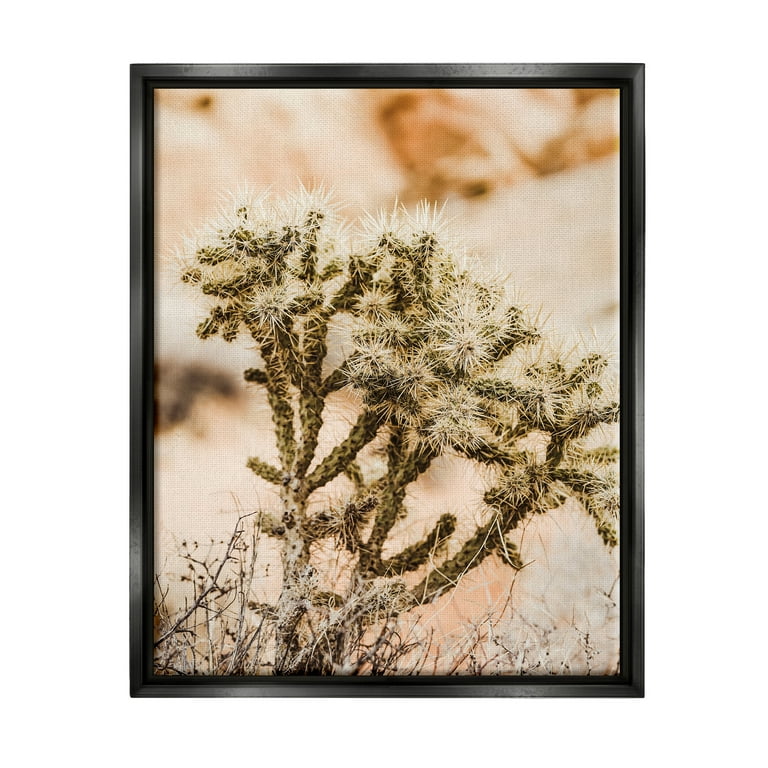The image showcases a close-up view of a plant that resembles a cactus, prominently displayed within a black picture frame. At the center and slightly towards the right of the picture, there are three to four upward-stretching, stalk-like stems of the cactus. Each stem has finger-like projections ending in dense clusters of white, bristly spikes. The background within the frame is blurred, featuring a beige-brown hue, particularly pronounced in the upper right corner, with a similar tone appearing faintly at the bottom. Surrounding the cactus, at the base of the image, are various smaller plants, grasses, and weeds, contributing to the natural setting. The overall composition directs attention to the spiky, intricate details of the cactus, contrasted against the out-of-focus, earthy backdrop.